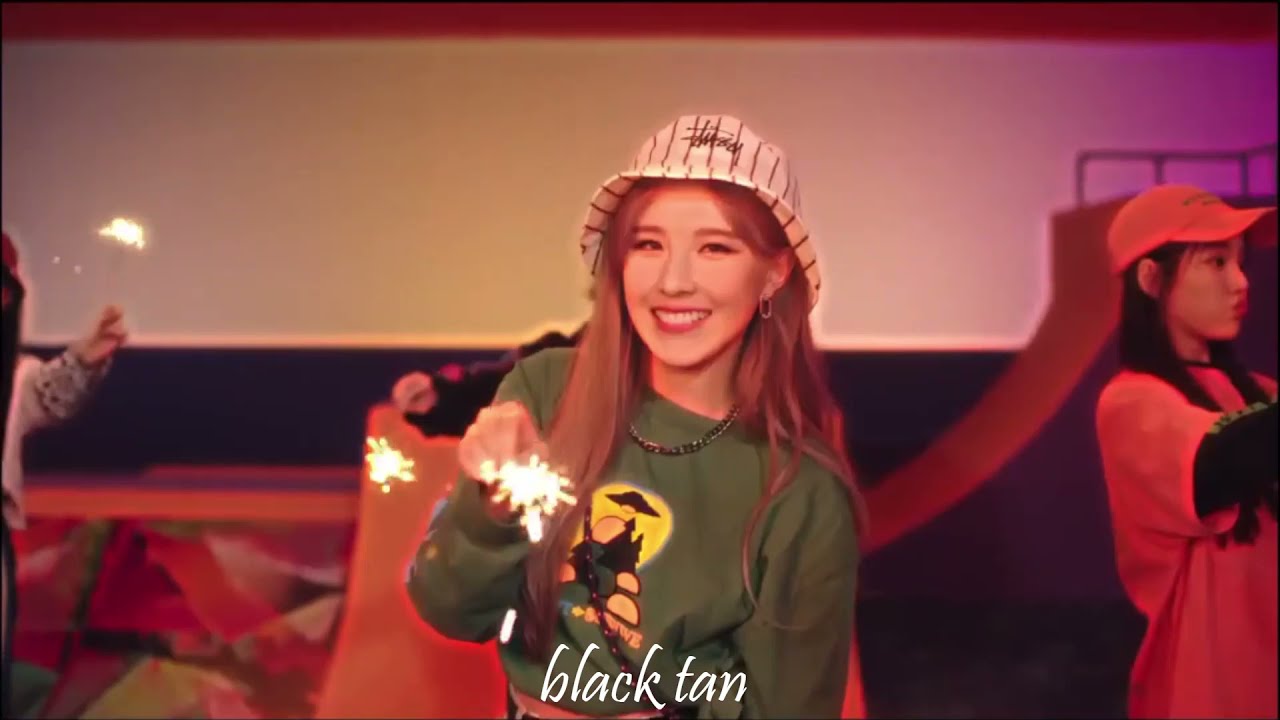In this vibrant image, a young woman with fair skin and long reddish-brown hair stands smiling at the center. She is wearing a green long-sleeved shirt adorned with an image featuring a person with a long black hat against a background of yellow and orange circles. She accessorizes with a black necklace, earrings, and a distinctive white Gilligan-style hat with vertical black stripes. Holding a sparkler in her hand, she looks directly at the camera. To her right is a young Asian woman with long black hair, wearing a red t-shirt over a black long-sleeved shirt, and an orange hat. She faces to her right, contributing to the festive atmosphere. Partially visible on the left is another woman, also holding a sparkler. The background features a brown half-pipe structure with visible rails in the upper right-hand corner, a white wall that fades into a black wall at the bottom. Text at the bottom of the image reads "black and tan" in white, hinting at the celebratory nature of the scene, possibly indoors during a New Year's celebration. Various colors such as brown, white, yellow, orange, red, green, and black enhance the lively setting.